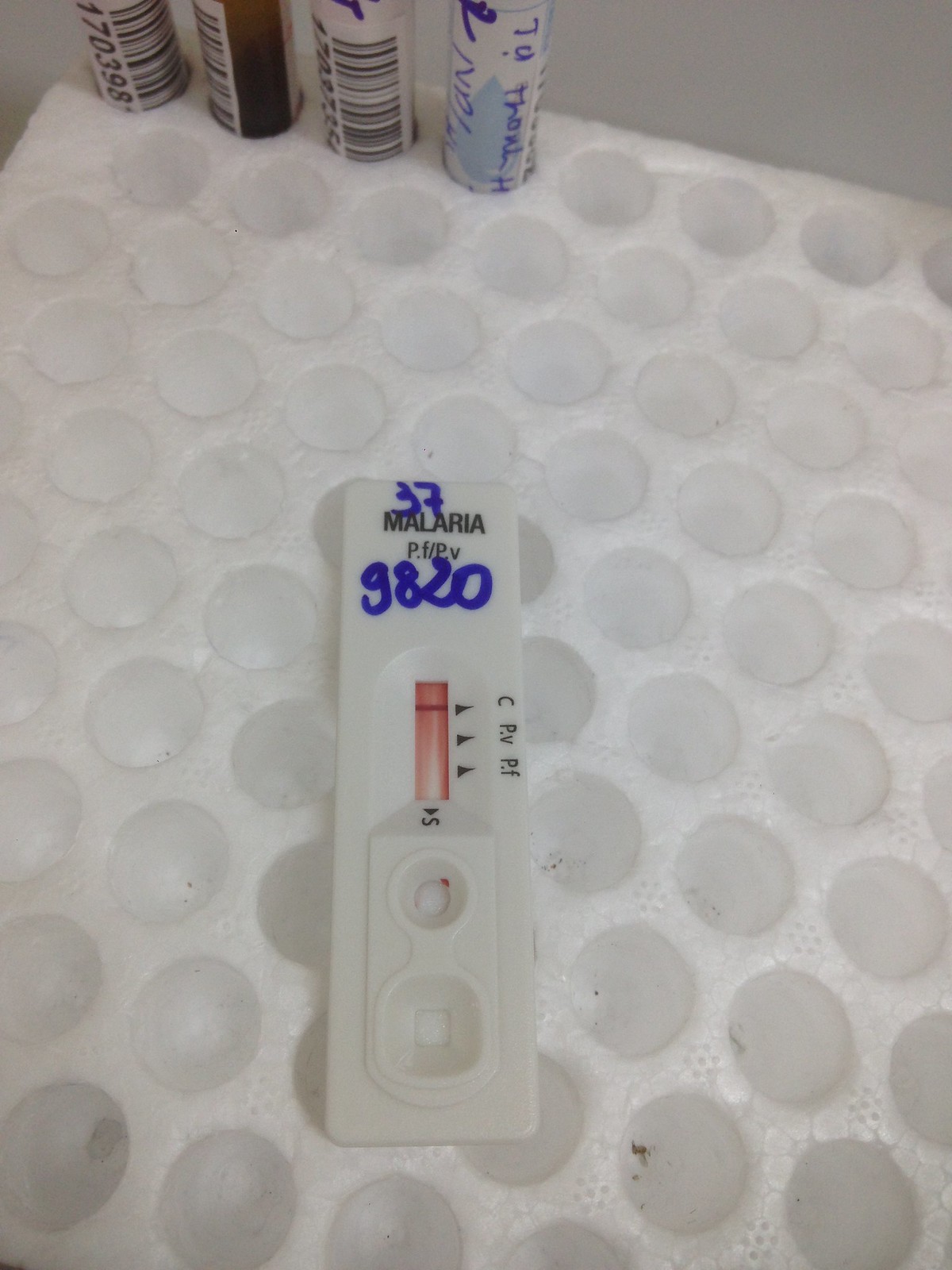The image depicts a laboratory setup for testing, featuring various components against a white wall background. At the forefront is a foam holder punctuated with numerous circular slots, specifically designed to secure sample vials, similar to those used for blood collection. In the upper left corner of the foam holder are four such vials. The first vial has a black-and-white UPC code labeled "170398". The adjacent vial has an opaque appearance with a brownish substance inside and also bears a UPC sticker, though its numbers are unclear. The third vial, positioned right next to the second, has an indistinguishable UPC code. The fourth vial stands out with a blue sticker, showcasing an image of a raindrop and blue text.

Towards the center of the image lies a malaria test strip labeled with "Malaria Test P.F./P.V." in black text. Handwritten blue marker inscriptions "379820" are also visible on the strip. The test strip has a red section marked with three right-pointing arrows, and near the top of this red area, two test lines labeled "C", "P.V." and "P.F." are visible. A horizontal red line cuts across the section. Towards the bottom of the strip, an "S" is marked, pointing downward toward a designated sample drop zone, featuring both circular and square areas.

The foam holder, while functional, displays signs of wear with visible specks of dirt scattered across its surface.